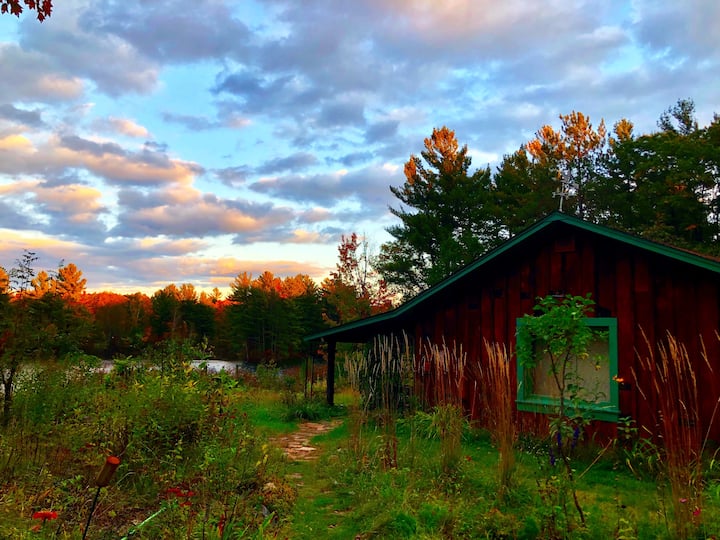This image features a small, older-style red wooden house with a green-trimmed sloped roof and a large green-framed window situated on the right side. The house is surrounded by an overgrown field of tall green grass, weeds, and brown reeds. In the background to the left, there is a pond partially visible through the foliage. The scene is framed by a mix of evergreen and deciduous trees, their upper branches adorned in a golden-orange hue from the setting sun. The sky occupies the upper portion of the image, presenting a blue canvas with clouds tinged in shades of orange, pink, and light purple, illuminated by the sunlight. This serene woodland setting captures both the tranquility of nature and the charming simplicity of rustic architecture.